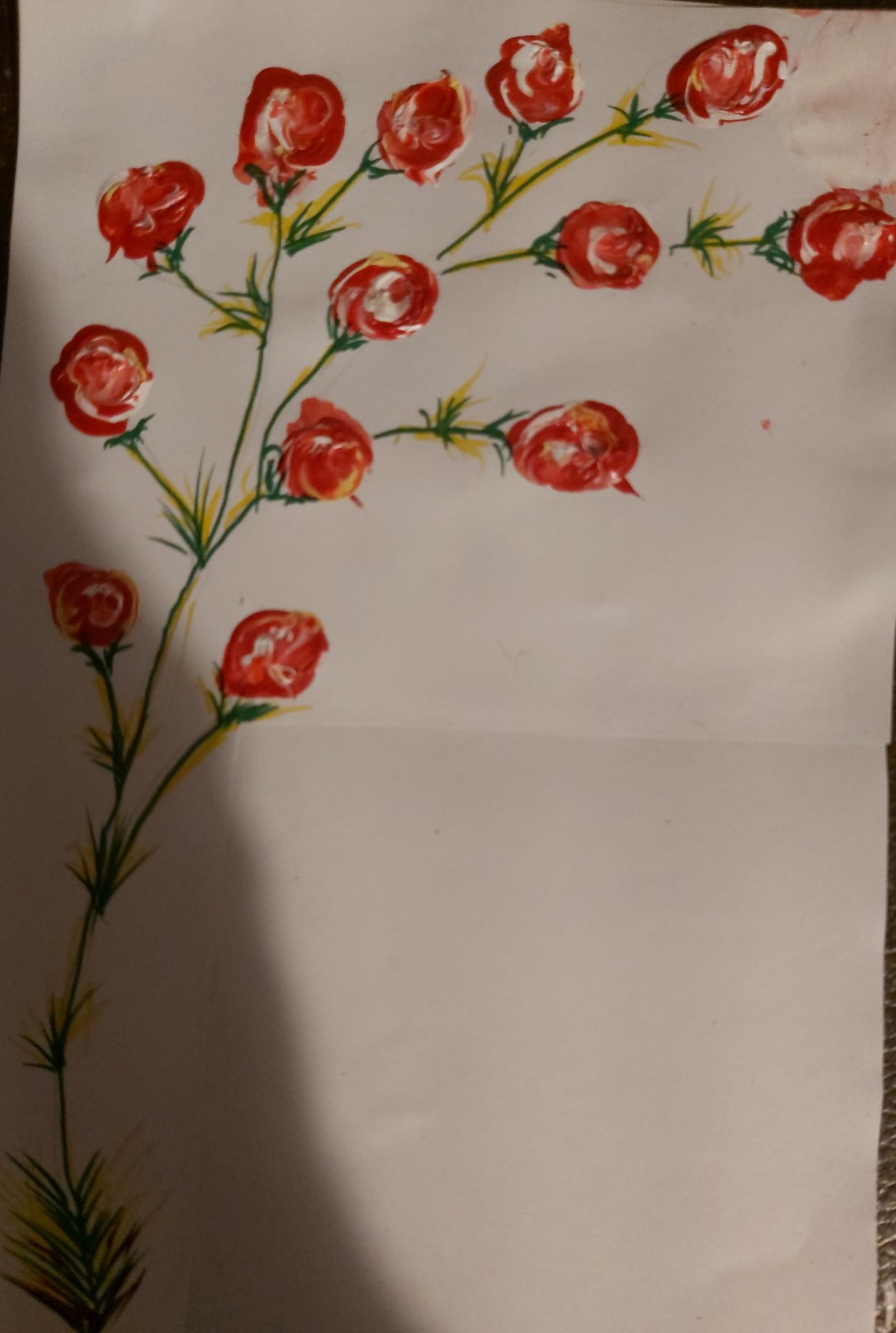This artwork features a beautifully detailed painting of flowers, resembling tulips or roses, on a pristine white piece of paper. The flowers are predominantly painted in vivid red hues, accentuated by intricate white swirling patterns that add depth and texture to the petals. A single green stalk with subtle yellow highlights emerges from the bottom left corner of the image, gracefully arcing upwards and to the left. This main stem branches out sporadically, with each branch typically supporting a solitary flower. Towards the top of the composition, the branching increases, showcasing a total of twelve exquisite red flowers that capture the viewer's attention with their vibrant coloration and delicate structure.